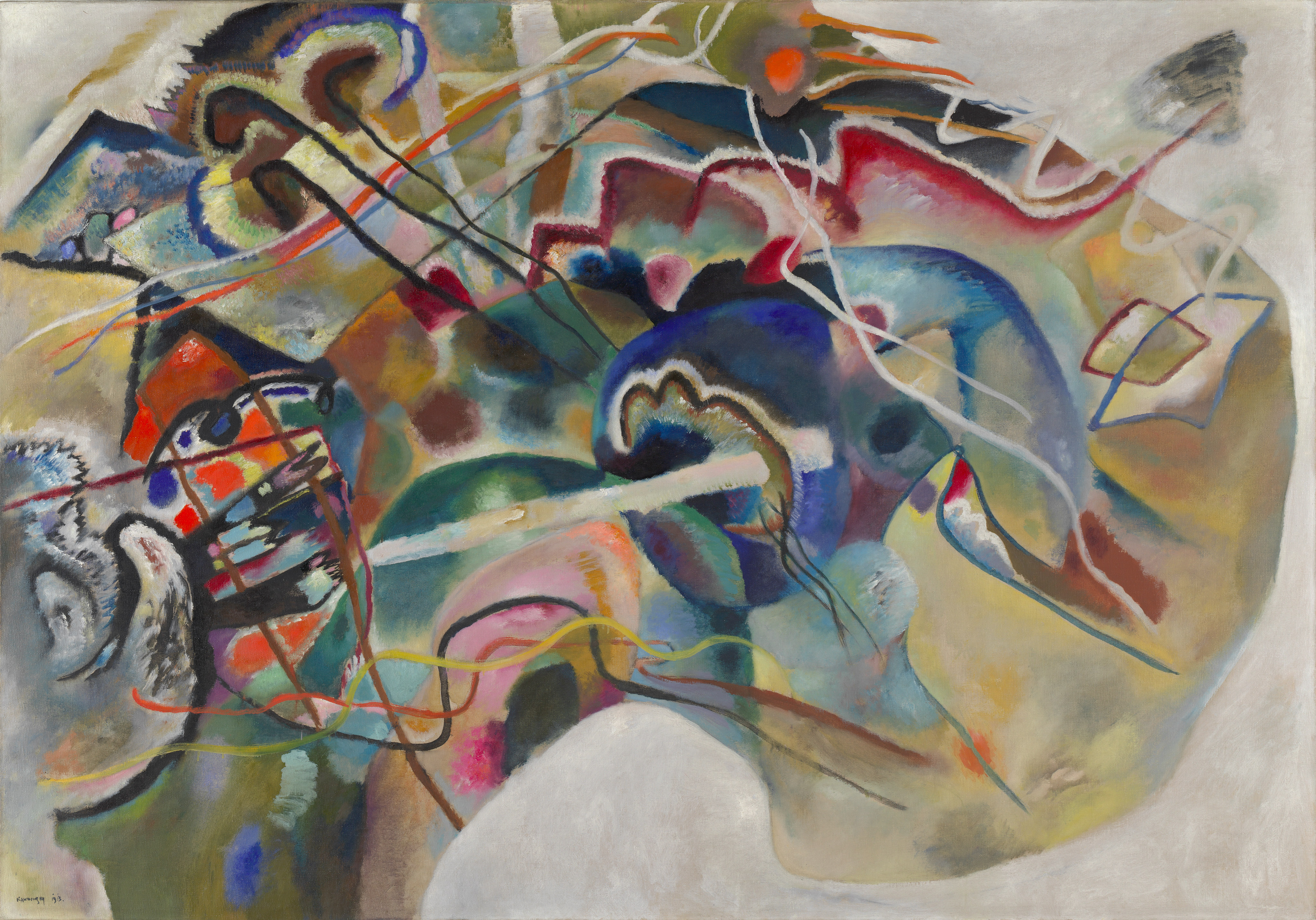The image showcases a vibrant, graffiti-style background teeming with splashes of colorful paint. Amidst the chaotic yet artistic backdrop, an abstract representation of a horse emerges. The horse's face is partially obscured by layers of paint but distinguished by a striking orange eye that contrasts sharply against the predominantly gray background. The horse appears to be facing towards the right side of the image, with its mouth and muzzle directed in that direction. The overall painting exudes an abstract and dynamic energy, blending elements of street art with surreal touches.